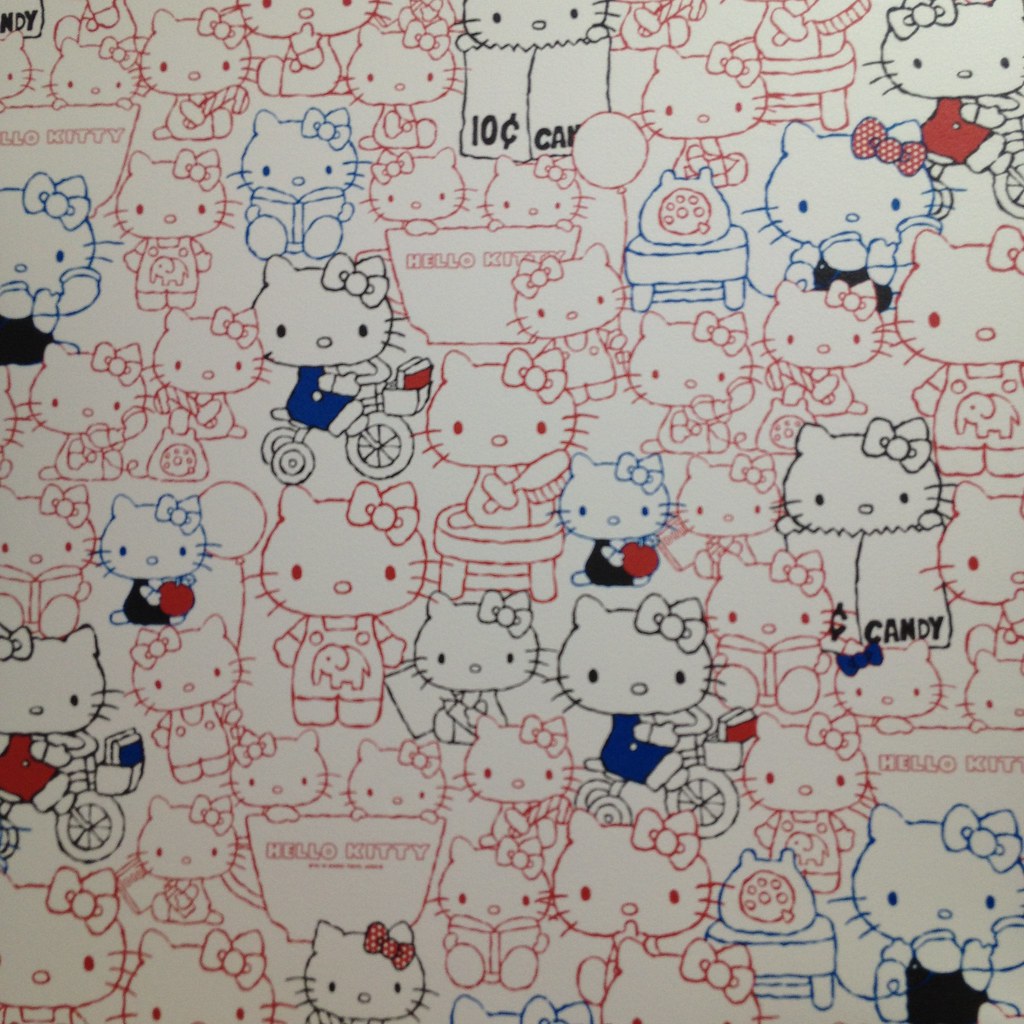The image depicts a densely populated scene of approximately 30 to 50 Hello Kitty illustrations on a white paper background. Each Hello Kitty is featured in various poses and activities, such as sitting, standing, riding a tricycle with books, using a rotary phone, holding an apple, and emerging from a candy bag labeled "10 cents candy." The illustrations are primarily outlined in red, but some are in black and blue, showcasing a variety of colors without being fully filled in. Notably, Hello Kitty can be seen in different outfits, including overalls with an elephant emblem and a bow. The images are distributed throughout the page, creating a vibrant and playful collage of Hello Kitty engaging in everyday activities, reminiscent of a detailed, multicolored ink drawing.